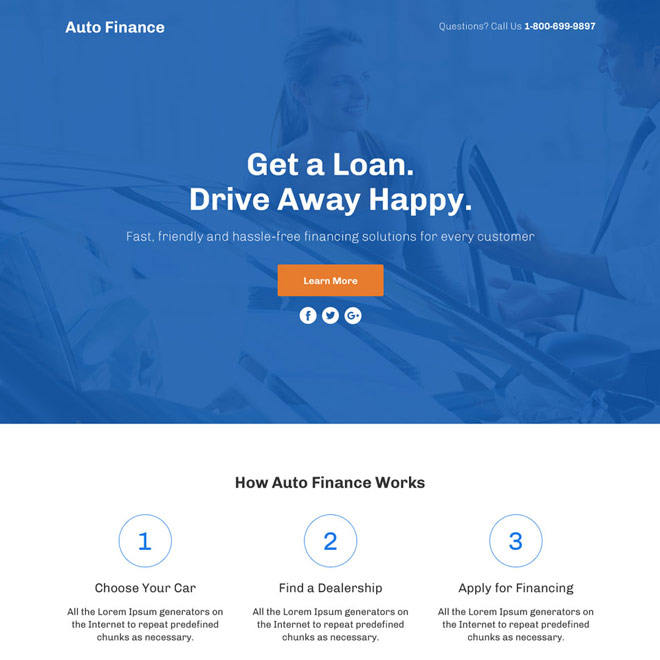Advertisement for an Auto Finance Company:

The advertisement features a clean and organized design set against a blue background, with various text elements in white and some in orange for emphasis. At the top, the company’s service is labeled "Auto Finance" in bold white lettering, followed by the phrase "Questions? Call us" in slightly smaller, but still white, text. The advertisement prominently displays a 1-800 phone number in white digits for easy readability.

An image in the background depicts a woman being sold a car by a gentleman, highlighting the customer interaction aspect of the service. Below this, the ad features the call-to-action phrases "Get a loan" and "Drive away happy." The latter is rendered in larger, more prominent white font to capture attention. 

Further down, the text reads: "Fast, friendly, and hassle-free finance solutions for every customer," emphasizing the company's customer-centric approach. An orange tab labeled "Learn More" in white text invites further engagement, accompanied by social media icons for Facebook, Twitter, and Google Plus (when it was still active), positioned underneath.

At the bottom segment, the phrase "How Auto Finance Works" is presented in black text. Beneath this, three blue numbered circles highlight the straightforward process:
1. Choose your car.
2. Find a dealership.
3. Apply for finance.

The advertisement effectively conveys a streamlined and customer-friendly auto finance process, yet notably does not mention the company's specific name, focusing instead on the generic service offered.